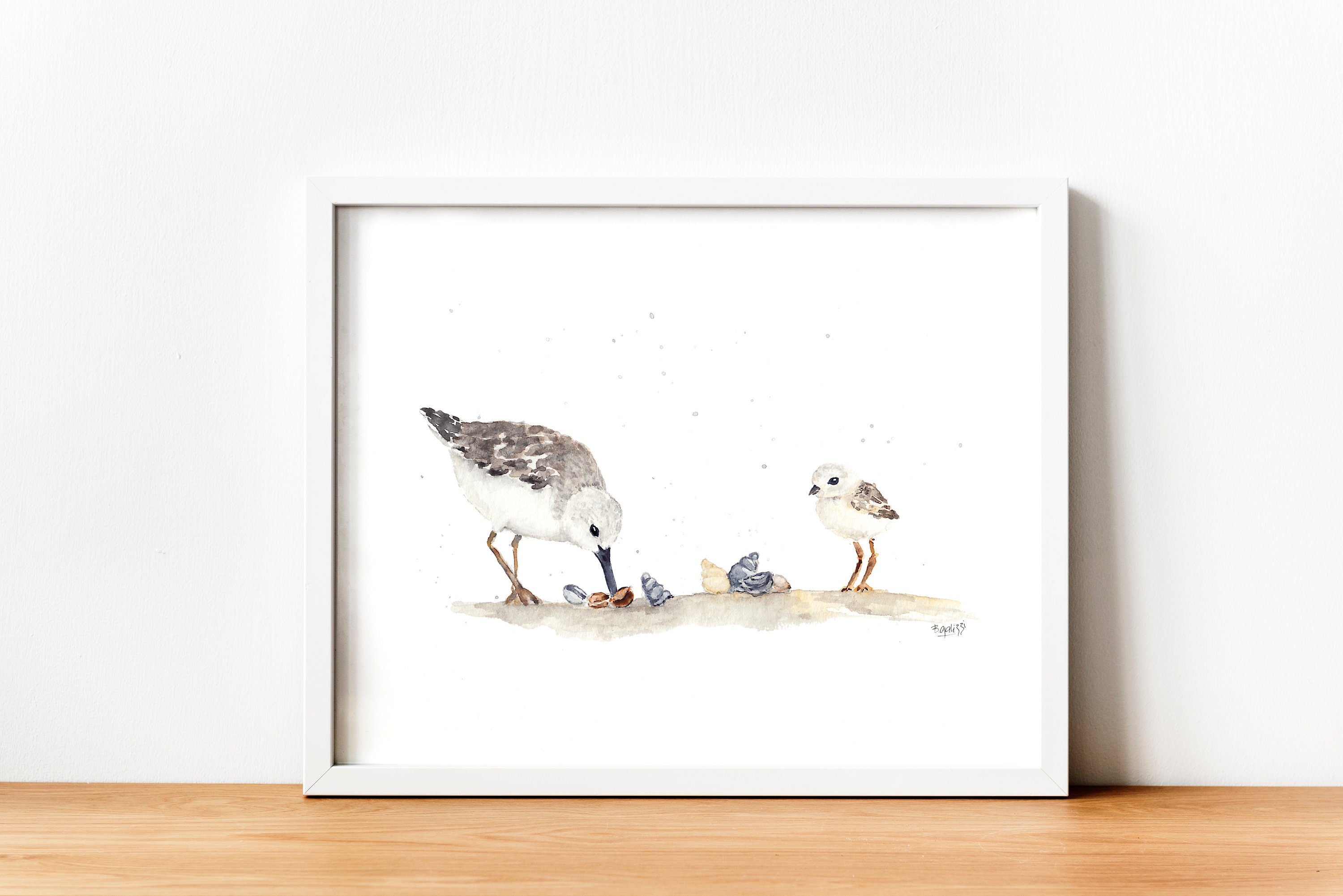The image depicts a white framed watercolor painting of two shorebirds, likely a sanderling or sandpiper, resting on a light wooden plank against a white wall. The adult bird is positioned on the left, beak pecking in the sand amid various snails and seashells, which range in shades of pale tan, gray, and brown. To the right, its young offspring observes, perhaps mimicking the adult's foraging behavior. The painting features a coastal color palette dominated by pale browns and the birds' distinctive orangish legs, against a stark white background with subtle gray speckles. The scene appears minimalistic, with the sand and figures fading into the distance. The artist's signature is located at the bottom right, beneath the baby shorebird.